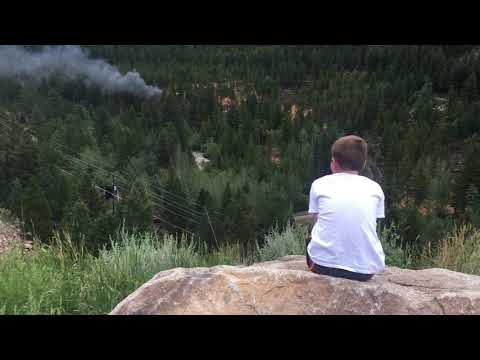A young boy with extremely short blonde hair sits on a large tan and gray boulder, wearing a white t-shirt and black pants. He gazes out over a sprawling, forested valley filled with a mix of bright green vegetation and numerous evergreen trees. Running through the bottom left corner of the valley are electric power lines. In the middle distance, a dark gray smokestack rises from the forest, with occasional white buildings visible through the trees. The scene suggests a hot summer day, and the boy appears to be enjoying the serenity and expansive view, perhaps part of a nature trail or national park.